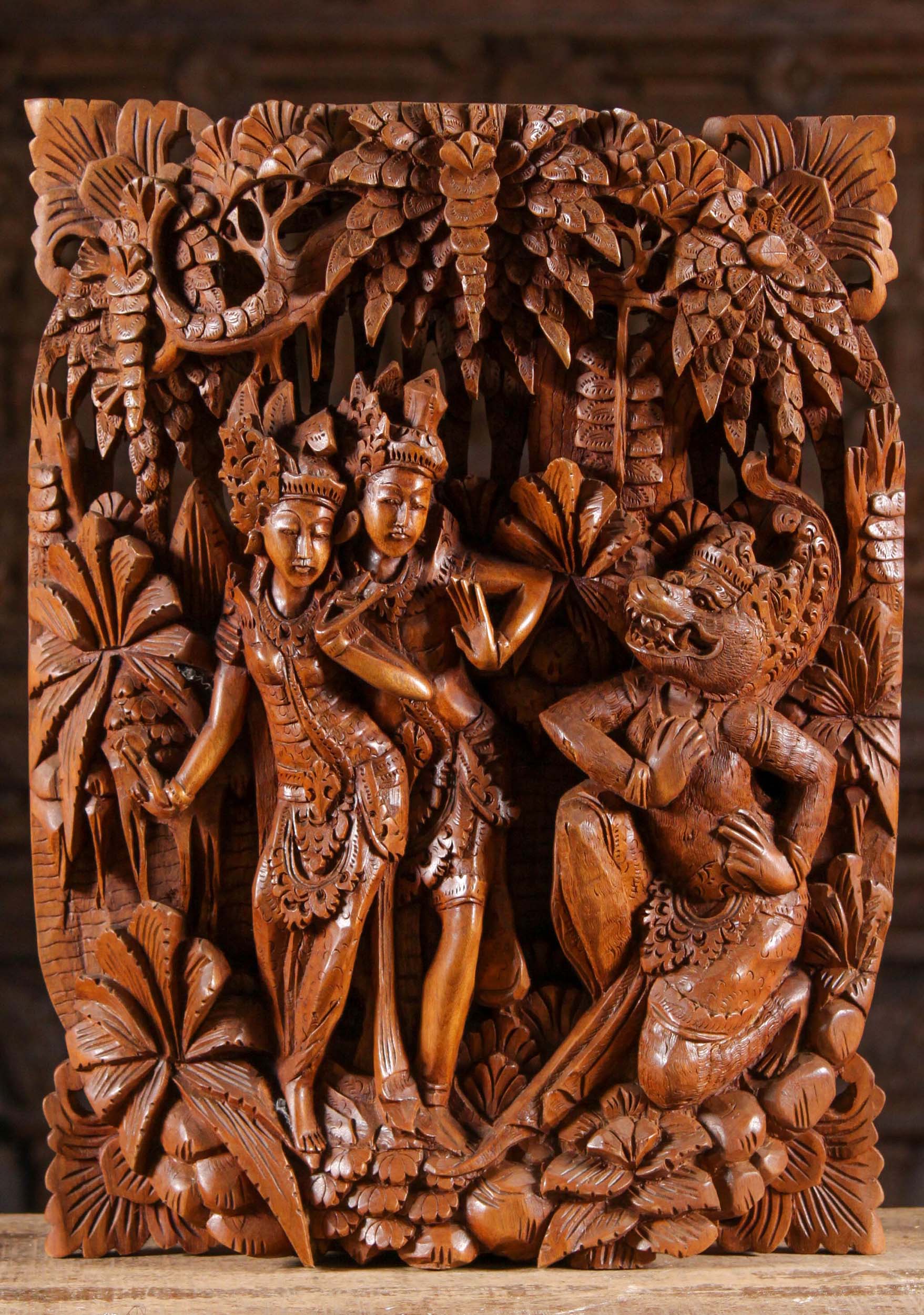This is a detailed photograph of an ornate Balinese wood sculpture, carefully carved from a warm brown wood and resting on a light-colored wooden table. The centerpiece features two slender Balinese women dancers, adorned with traditional headdresses. They are portrayed in dynamic dance postures, with arms raised and hands bent, one of the hands resembling a peace sign. The women's bodies have intricate palm leaf designs, and they are surrounded by carvings of ferns and various foliage that flare out from the sculpture’s rectangular base. To the right of the dancers is a figure of a humanoid creature with the body of a man and the head of a fearsome creature, described variably as a wolf or a Komodo dragon, sporting sharp teeth and an open, snarling mouth. This creature, depicted kneeling on one knee with one hand on its heart and the other on its hip, wears a crown, enhancing its god-like presence. The entire sculpture is enriched with three-dimensional carvings of palm tree leaves, flowers, and cornucopia, combining to create a rich and detailed piece of art with a deep brownish-red coloration.